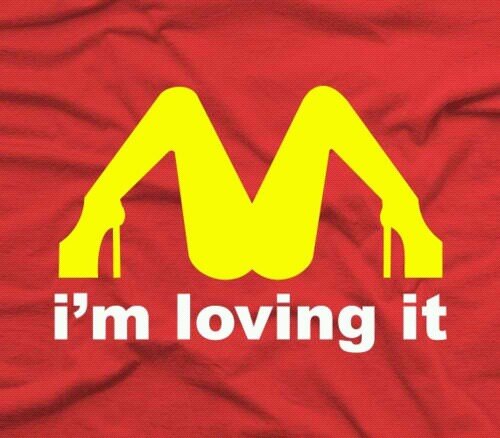The image features a bright cherry red fabric that appears to be a t-shirt material. Prominently displayed on this fabric is a creative and cheeky logo resembling the iconic McDonald's "M". Cleverly integrated into the "M" design are the yellow silhouettes of a woman's legs and bottom, positioned in a way that her knees form the top arches and the space between her legs forms the central dip of the "M". She is depicted wearing high heels, further accentuating the playful nature of the design. Below the "M", in white font, is the familiar McDonald's slogan "I'm loving it", adding an extra layer of humor with a suggestive twist. The fabric itself is not entirely smooth, with slight undulations indicating the natural texture of the material. The striking combination of bright yellow, red, and white colors ensures the logo stands out vividly against the red background.